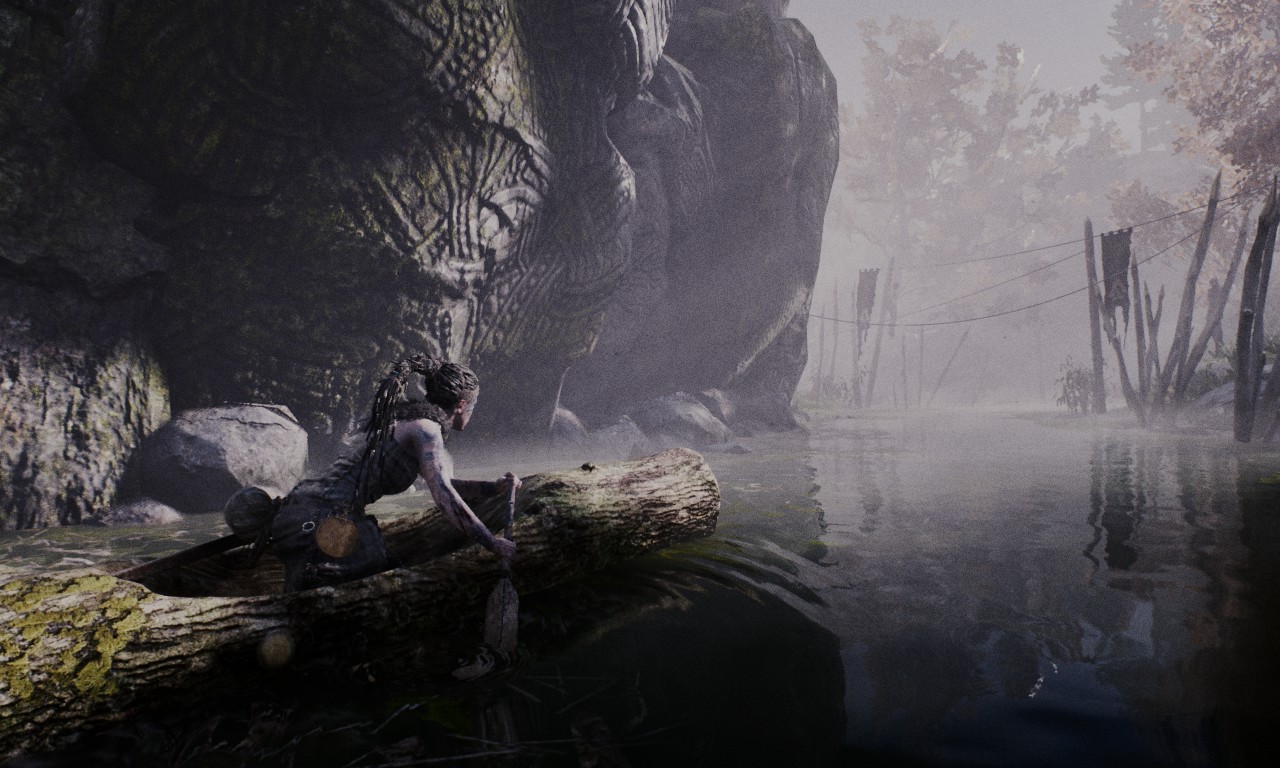A solitary figure is seated in a carved-out log boat, hunched forward in intense concentration. Dressed in a tank top and tight pants, a distinctive brown circle marks the fabric on their backside. They hold a stick that widens at the bottom, poised for navigation. Their hair is neatly pulled back into a ponytail. The boat glides through dark, haunting waters enveloped by dense fog. In the distance, a series of spikes protrude from the water, connected by a cable draped with cloth, stretching to either side of the misty expanse. On the left, rocks with intricate carvings—lines, squares, and diamonds—rise from the water. The somber scene is further accentuated by the presence of barren, dead trees in the background, under a sky punctuated by what seems to be a rocket ascending into the atmosphere.